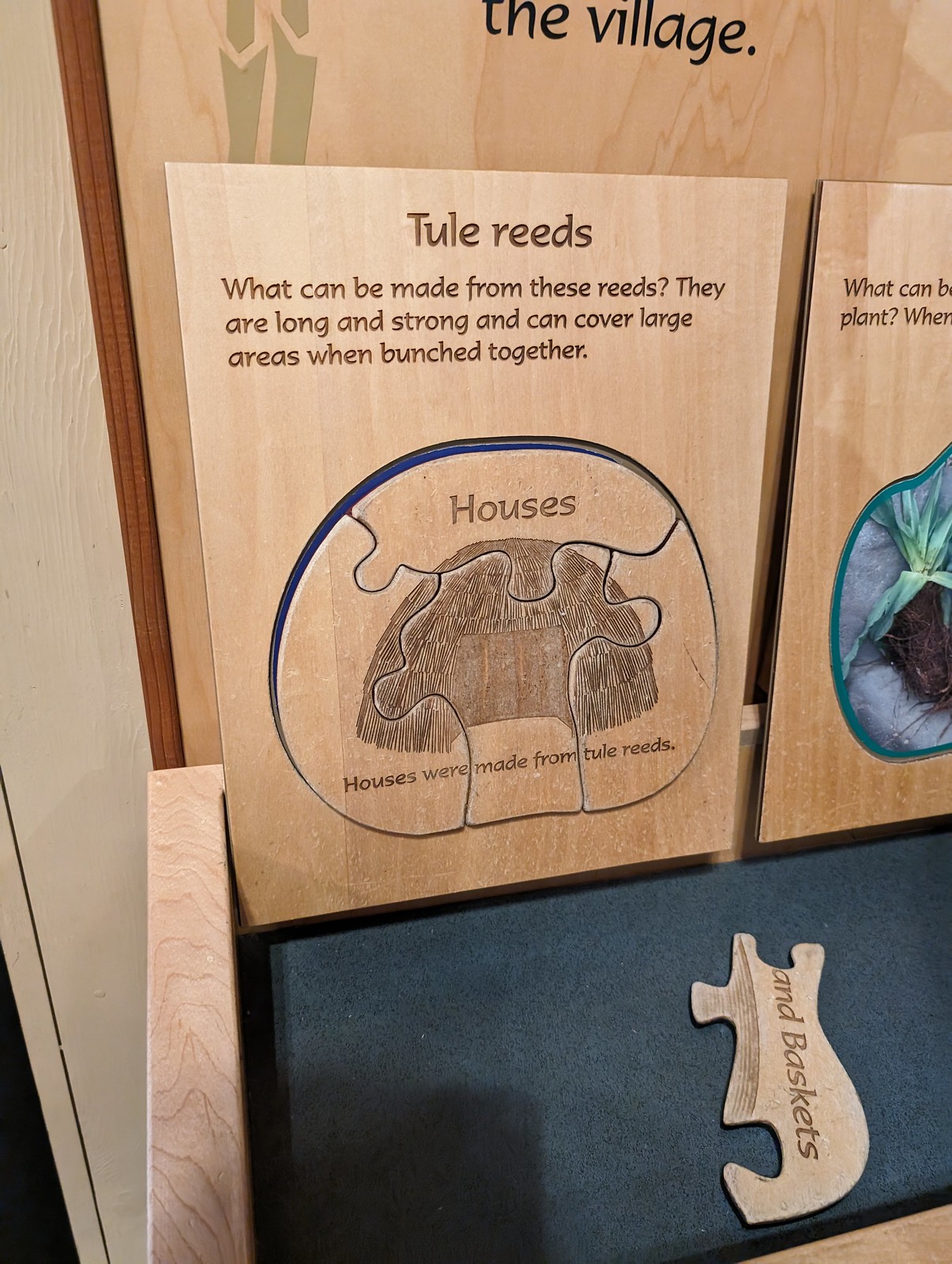The image depicts a detailed and informative display featuring a wooden jigsaw puzzle, possibly part of a museum exhibit. The centerpiece is a prominent wooden placard that's leaning against several smaller wooden placards. The main placard reads "The Village" at the top, followed by the text "Tool Reeds" carved into it. Beneath this, an informative description explains: "What can be made from these reeds? They are long and strong and can cover large areas when bunched together."

In front of the placards on a blue velvet shelf, there is a wooden jigsaw puzzle comprising four pieces. One piece highlights the word "houses," with further details about tool reeds specifying that "houses were made from tool reeds; they were long and strong and can cover large areas when bunched together." Another piece illustrates a hut made from bundled tool reeds, emphasizing their use in historical construction methods. Additionally, a separate puzzle piece labeled "and baskets" suggests potential uses for tool reeds beyond building houses. This engaging display appears to be designed to educate viewers, possibly children, on traditional building materials and methods.